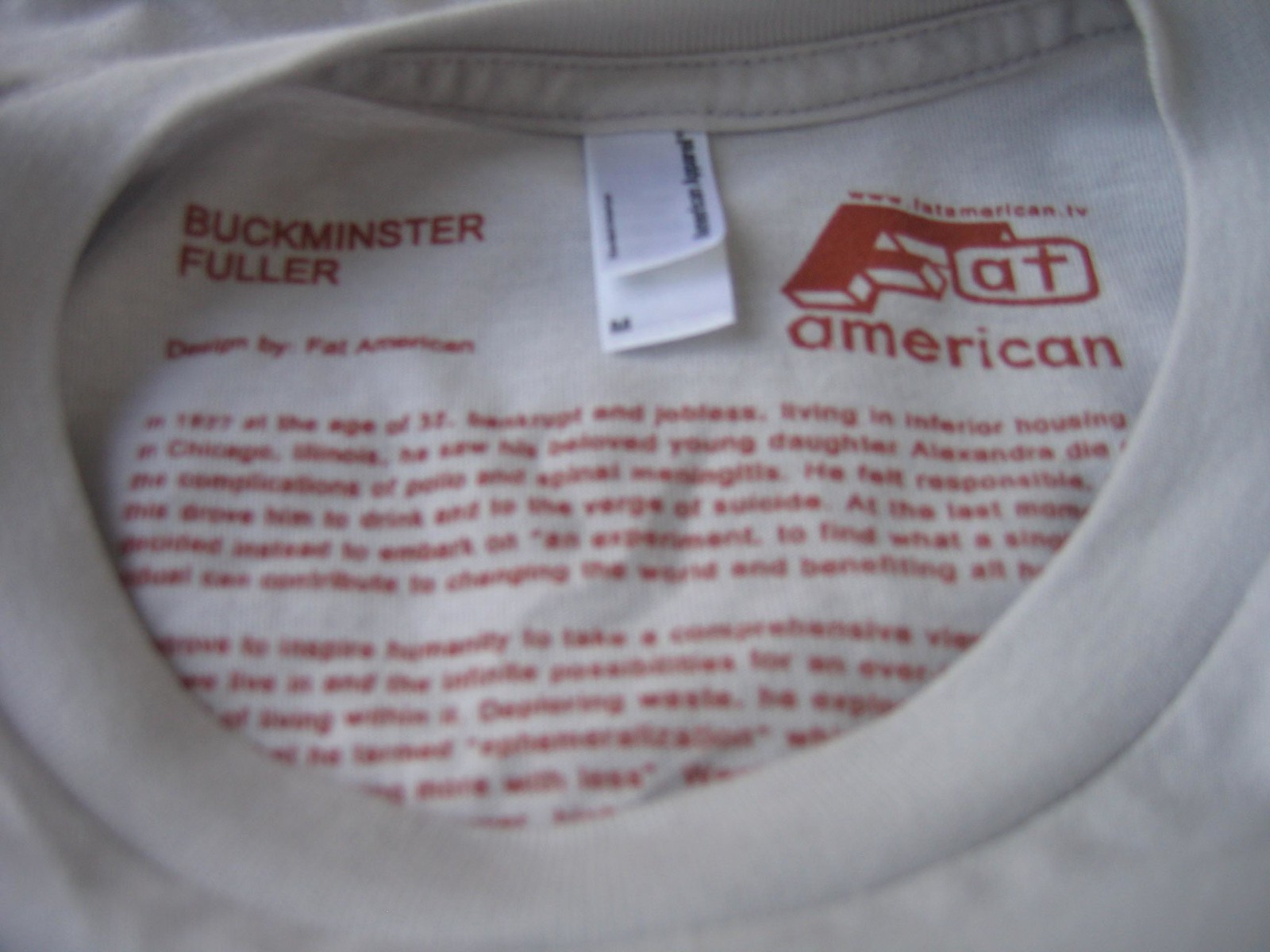This image showcases the neckline of a round-neck, white shirt featuring a ribbed collar. The interior view of the shirt reveals an abundance of red printed text, most of which is illegible. However, prominently displayed is the name "Buckminster Fuller," likely indicating the manufacturer. A white label with two sections hangs down, with the size marked as medium. To the right of the label, a large red "F.A.T. American" is visible, which appears to be part of the maker's logo.